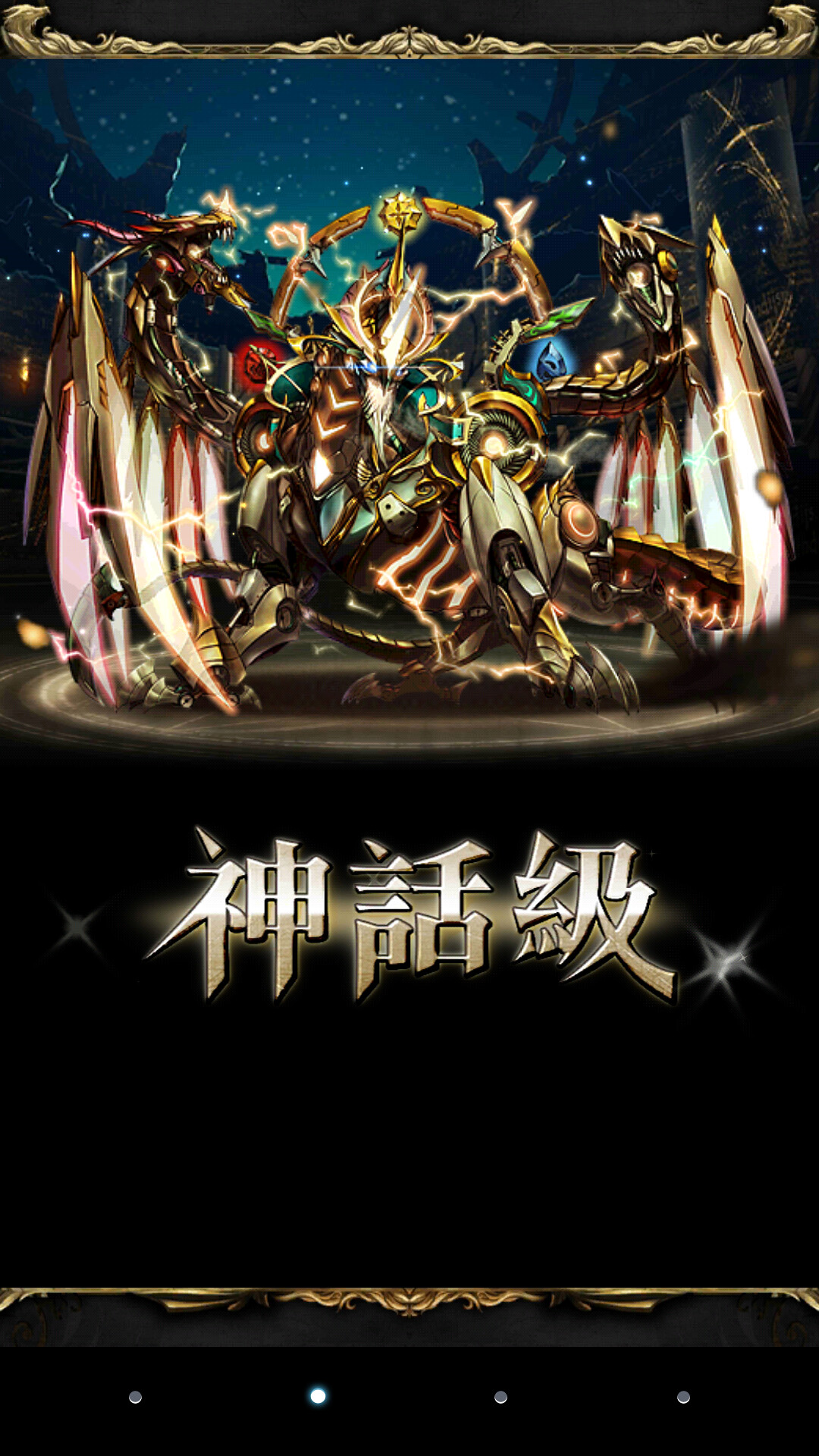The title screen of the game prominently features a colossal bird-like robot with dual dragon heads emerging from its sides. The creature boasts robotic, clawed legs and expansive wings composed of vibrant streams of light. Its dynamic presence is enhanced by a backdrop of stars, adding a sense of cosmic grandeur. Dominating the lower half of the screen is the game's title, displayed in shiny gold Chinese characters, which are further accentuated by a radiant golden glow. At the bottom of the image, four silver buttons are neatly aligned.